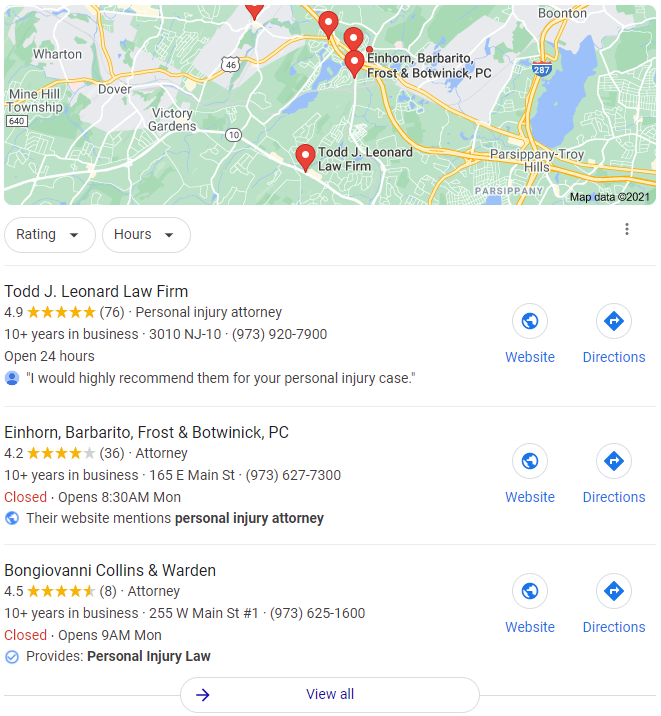The image displays a Google Maps-like interface featuring a green landmass with a network of white lines indicating roads and yellow lines denoting highways. Several locations are prominently marked on the map, such as Parsippany, Troy Hills, Boonton, Dover, Victory Gardens, Wharton, and Mine Hill Township. Multiple red markers indicate specific places, with detailed listings provided below the image.

The first listing is for the Todd J. Leonard Law Firm, which has a 4.9-star rating from 76 reviews and identifies as a personal injury attorney with over 10 years in business. The firm is available 24 hours and has a listed phone number. A testimonial reads, "I would highly recommend them for your personal injury case." There are two buttons adjacent to this listing: "Website" and "Directions."

Below this, the second listing is for Einhorn, Barbarito, Frostwick, and Botwinick PC. The firm is currently closed but also boasts over 10 years in business. The address is provided, and the firm's website mentions its specialization in personal injury law.

The third listing is for Bon Giovanni Collins and Wharton, which also shows reviews and is presently closed. This firm is noted for providing personal injury law services.